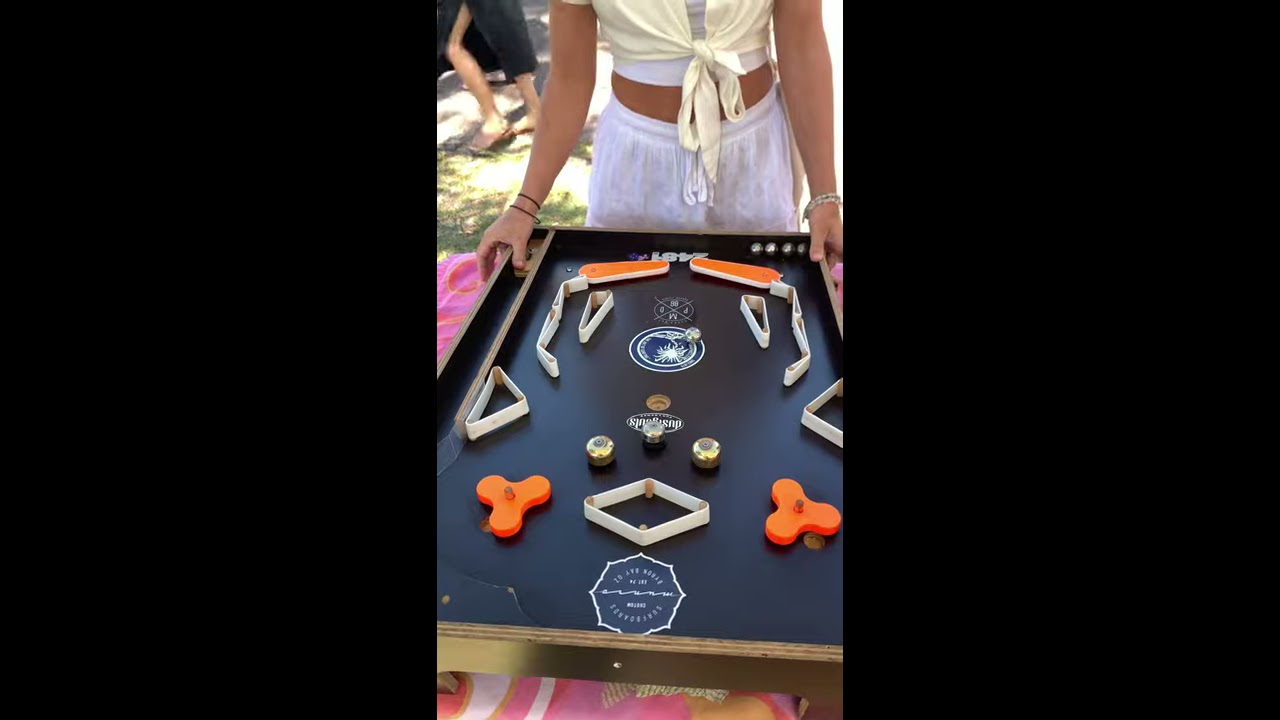This image captures a photograph framed between two black bands, focusing on an intricately designed panel reminiscent of a pinball machine. The panel, a 3D collage of paper, features symmetrical arrangements of flippers, bumpers, and other elements typical of pinball patterns, yet it appears more like an artistic piece without a glass top. In the foreground, a girl stands beside the table, holding its sides rather than playing. She is dressed in white pants, a white t-shirt, and a tied white top, accessorized with bracelets on her arms. The table itself sports a pink, white, and yellow tablecloth, and its black base displays a firework logo. In the background, partially cut off, another person is visible, possibly holding a plaque, while a second girl in a black dress with a slit walks by, suggesting the scene might be part of an outdoor gathering or backyard party.